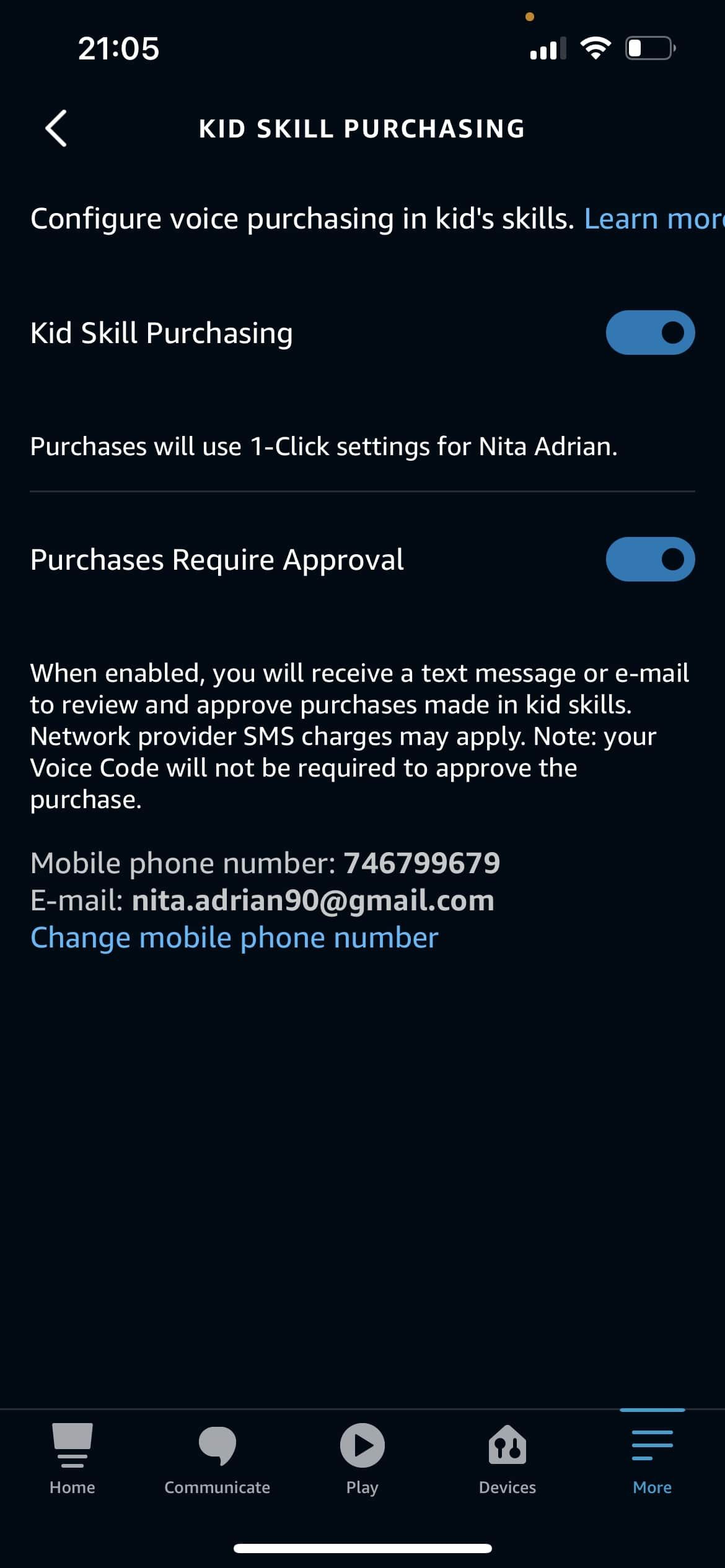### Caption

This detailed image shows a cell phone screen with a predominantly black background displaying white text interspersed with blue links. At the top left corner, the time is displayed as 21:05. The top right corner features icons indicating cell signal strength, wireless connection, and battery status.

Below these indicators, on the top left, there is a small arrow pointing left. Adjacent to this arrow, in all capital letters, the text reads "KidSkill Purchasing." The next line reads "Configure Voice Purchasing in KidSkills" followed by a blue link labeled "Learn More."

Further down, the screen reiterates "KidSkill Purchasing," indicating that this option is enabled. The text explains that purchases will use one-click settings associated with Anita Adrian and that these purchases require approval. This feature is confirmed to be enabled. When enabled, the user will receive a text message or email to review and approve purchases made in KidSkills, though SMS charges from the network provider may apply. It is noted that the user's voice code will not be required to approve purchases.

The current mobile phone number listed is 746-799-679, and the email provided is nita.adrian90@gmail.com. There is a blue link titled "Change Mobile Phone Number" for user convenience.

At the bottom of the screen, there are five icons labeled with corresponding functions: "Home," a speech bubble labeled "Communicate," a play button labeled "Play," "Devices," and a final option labeled "More."